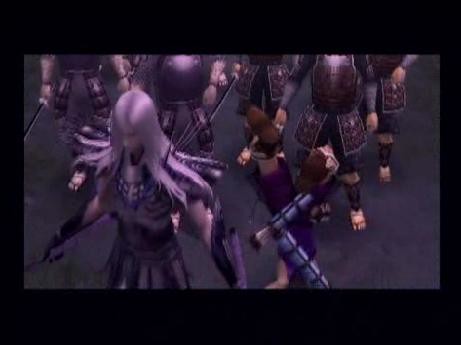This is a computer-generated image, a screenshot from a computer game. The scene is framed by a black box border. Centrally featured is a tall warrior with long, flowing white hair, parted down the middle, suggesting a male figure. This main character is outfitted in gleaming silver battle armor with additional dark shoulder pads, extending broadly over the shoulders. The forearms are also protected with silver armor, equipped with large gauntlets that have wrist shields, detailed with black and purple accents. A distinctive silver battle skirt and silver shoulder piece complete the ensemble. The warrior holds a sword in their right hand. Surrounding this central figure, in the background, are several other soldiers. These soldiers are clad in armor that varies from silver to a coppery-brown tint, with some appearing barefoot. Notably, a purple-like figure stands beside the silver-haired warrior, adding more intrigue to the scene. The background remains mostly black, emphasizing the armored characters in the foreground.